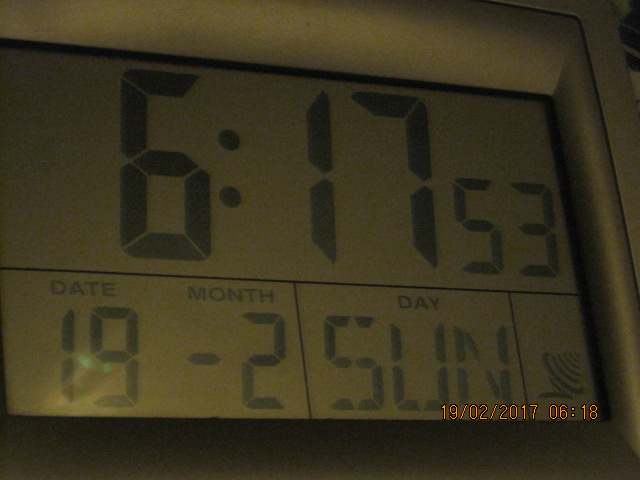This image showcases a digital clock with a large, easy-to-read display. The clock prominently shows the time as 6:17:53. In addition to the current time, it provides the date information, displaying "19" for the date and "2" for the month, indicating February 19th. The day of the week, "Sunday," is also visible. In the bottom right corner of the screen, there is text in orange that reads "19.02.2017" and "06.18," corroborating the date and time information displayed by the clock.